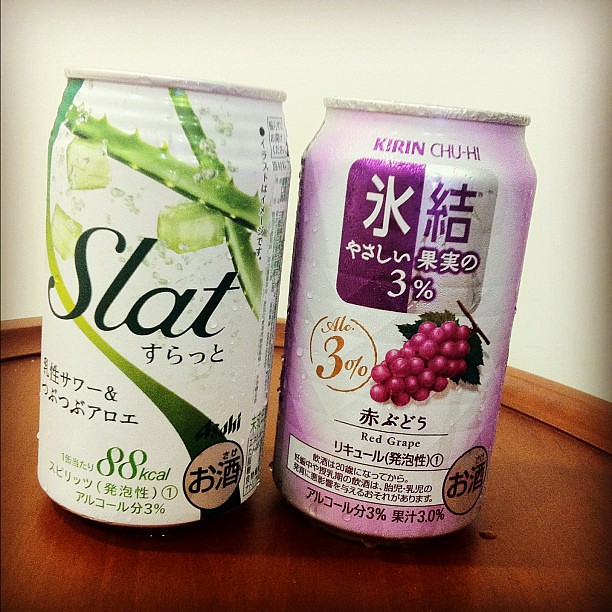This photograph captures a minimalist scene with a pristine white wall as the backdrop, juxtaposed against a rich, coffee-colored wooden surface. On this surface sit two soda cans, both of which stand out in their unique designs and cultural detailing.

Starting from the left, the first soda can is predominantly white, adorned with an artistic splash of coffee-colored liquid that seems to cascade across the front. Animated ice cubes, matching the hue of the liquid, appear to be dynamically shooting into the air, adding an element of excitement to the can's design. Below this vivid imagery, the can features the word "SLAT" in bold black font, accompanied by Asian characters underneath. At the very bottom, the calorie content is noted as "88 K-Cal" in a subtle brown color.

Moving to the right, the second can is also primarily white but is distinguished by a striking blue label. The label showcases a graphic of lush, purple grapes, lending a fresh and fruity visual appeal. The top of the can reads "Kirin Chuhi" in English, while the rest of the text is presented in Asian script, enhancing its exotic allure.

Overall, the image portrays a blend of cultural aesthetics and vibrant design elements, set against a simple yet elegant background.